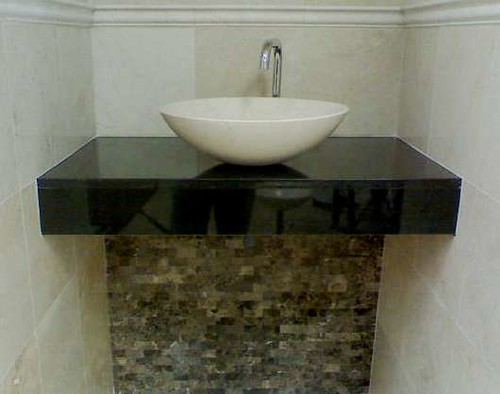This photograph captures a sleek, built-in black vanity with a glossy, lacquered finish, viewed directly from the front. Atop the vanity sits a pristine, white bowl-style sink, complemented by an elegant silver faucet arching over it. The bowl is relatively small and casts a faint shadow underneath. Surrounding the vanity is a striking wall of multicolored tiles in shades of brown, gray, and black, adding a touch of modern sophistication. The entire setup is nestled within a three-sided enclosure of large, cream-colored tiles, which are accentuated by a single horizontal strip of thin, narrow white tile running across the upper portion of the walls. The vanity itself is devoid of drawers, emphasizing a minimalist design aesthetic.